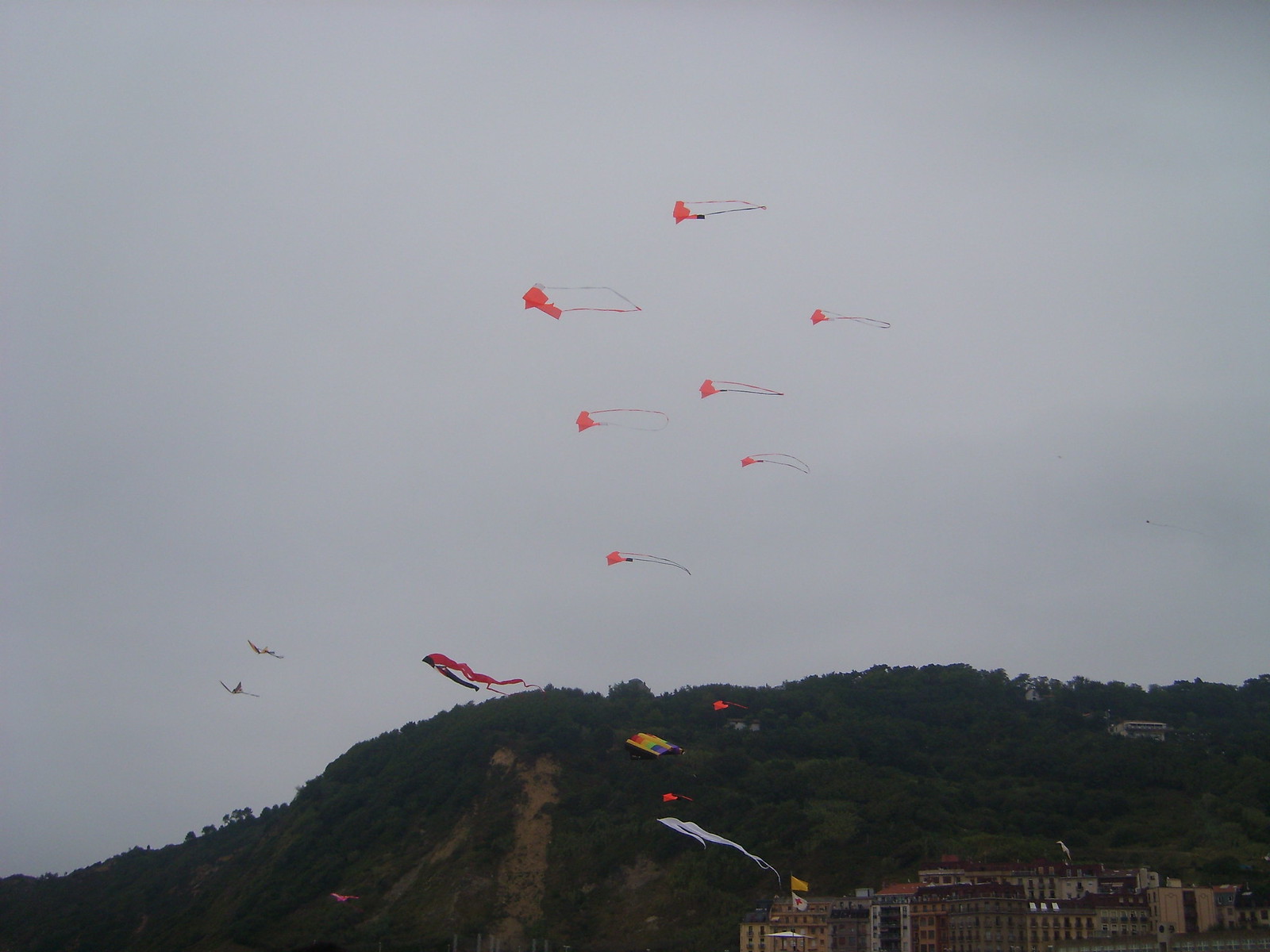The image showcases a sky full of kites flying over a lush, green hillside. The sky is a thick, uniform gray with no distinct clouds visible. Most of the kites are an orangish-pink color, with a particularly notable group of seven flying in close formation. These kites have shorter tails compared to some of the others. Below this group, a few additional kites are seen closer to the hills, including a distinctive red kite with a very long tail. The hillside is steep with tree-covered bluffs and a scattering of houses nestled among the trees. To the right, there is a large multi-story building, possibly a hotel or university complex, silhouetted against the overcast sky. There are at least 20 kites in total, including bright blue, white, red, and multicolored kites, their longer tails streaming to the right, indicating a windy day. The scene captures a serene yet dynamic moment, possibly a kite festival, with the vibrant kites standing out against the muted backdrop.